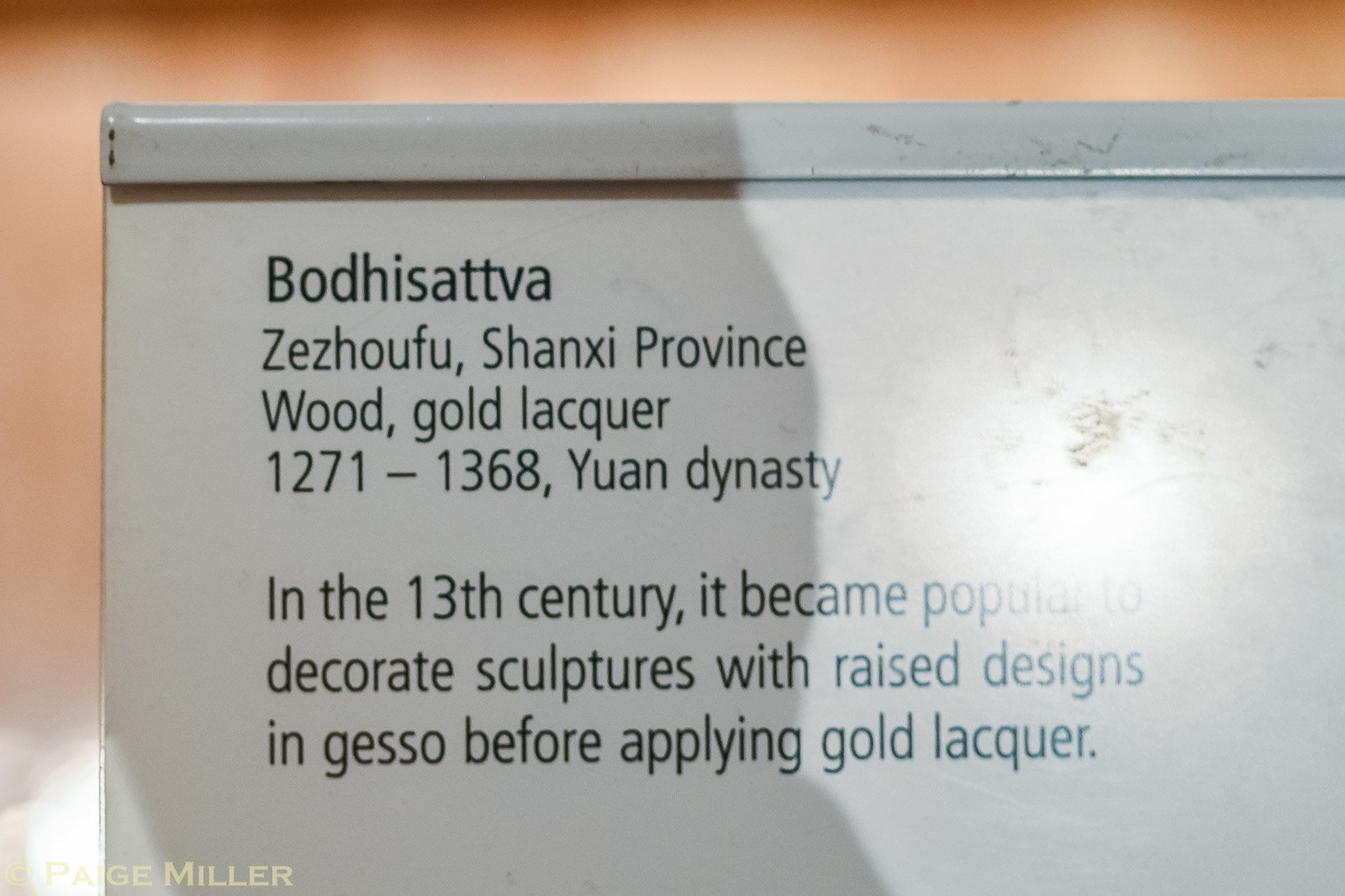The image depicts a close-up of a descriptive placard set against a tan or orange-brown background, likely within an indoor setting such as a museum. The placard itself, situated centrally within the frame, appears gray or metallic and contains black text that provides detailed information about an artifact. The text reads: "Bodhisattva, Zezhofu, Shanxi Province, Wood, Gold Decor, 1271 to 1368, Yuan Dynasty." It mentions that in the 13th century, it became popular to decorate sculptures with raised designs in gesso before applying gold decor. Additionally, there is an attribution mark at the bottom left corner of the image, stating "Paige Miller." The image features hues of tan, gray, white, black, and shadows on the left side.